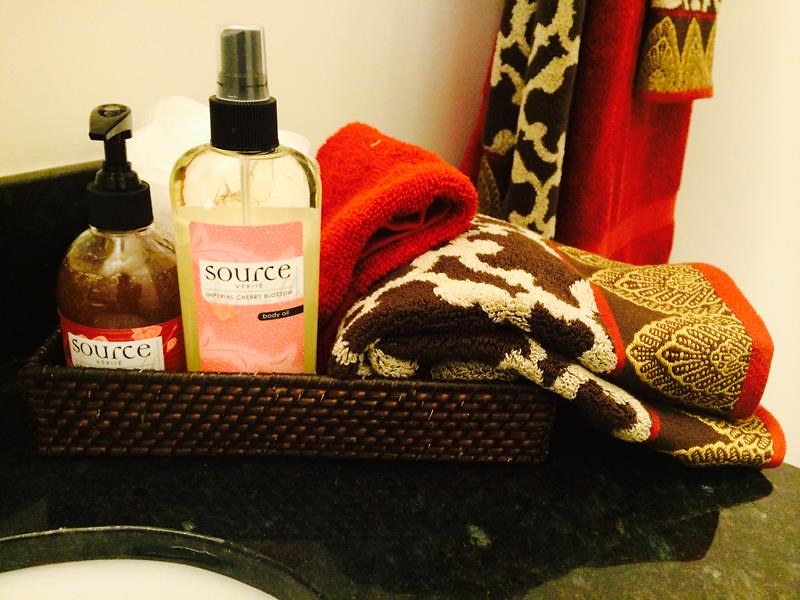A black wicker basket sits atop a pristine bathroom sink, creating a striking contrast. Inside the basket lies a neatly folded red bath towel, its vibrant hue juxtaposed with a smaller, intricately folded brown and white patterned face towel. The face towel features a striking red border and subtle yellow embroidery detailing at the front. Centrally placed within the arrangement is a spray bottle with a pink label bearing the word "Source" and the enticing fragrance description, "Cherry Blossom." To the left of this centerpiece stands another "Source" labeled bottle, distinguished by its red background and convenient pump-top design. This setup combines functionality with a touch of elegance, offering a serene and organized bathroom aesthetic.